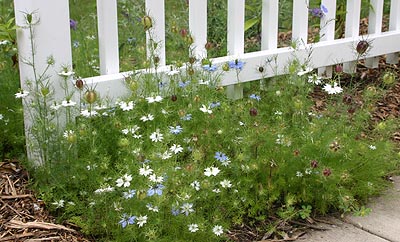This is a detailed close-up photograph of a bed of flowers taken outside during the day. The flower bed is covered with brown mulch and situated in front of a white picket fence and a concrete sidewalk. The fence spans the left side of the image, showing only the bottom several inches, where vertical slats are connected by a horizontal board at the base. The flowers include a mix of predominantly white and cyan blue petals, with some intertwined in the center of the bed, creating a vivid contrast. To the left, there's a concentration of white flowers, while the right side features three prominent white flowers and a few red ones, probably wilting blue or white flowers. Scattered green leaves add to the scene’s natural setting, which appears slightly disordered, suggesting perhaps a blend of wildflowers or weeds. Despite the untidiness, the image captures a charming and lively garden scene.